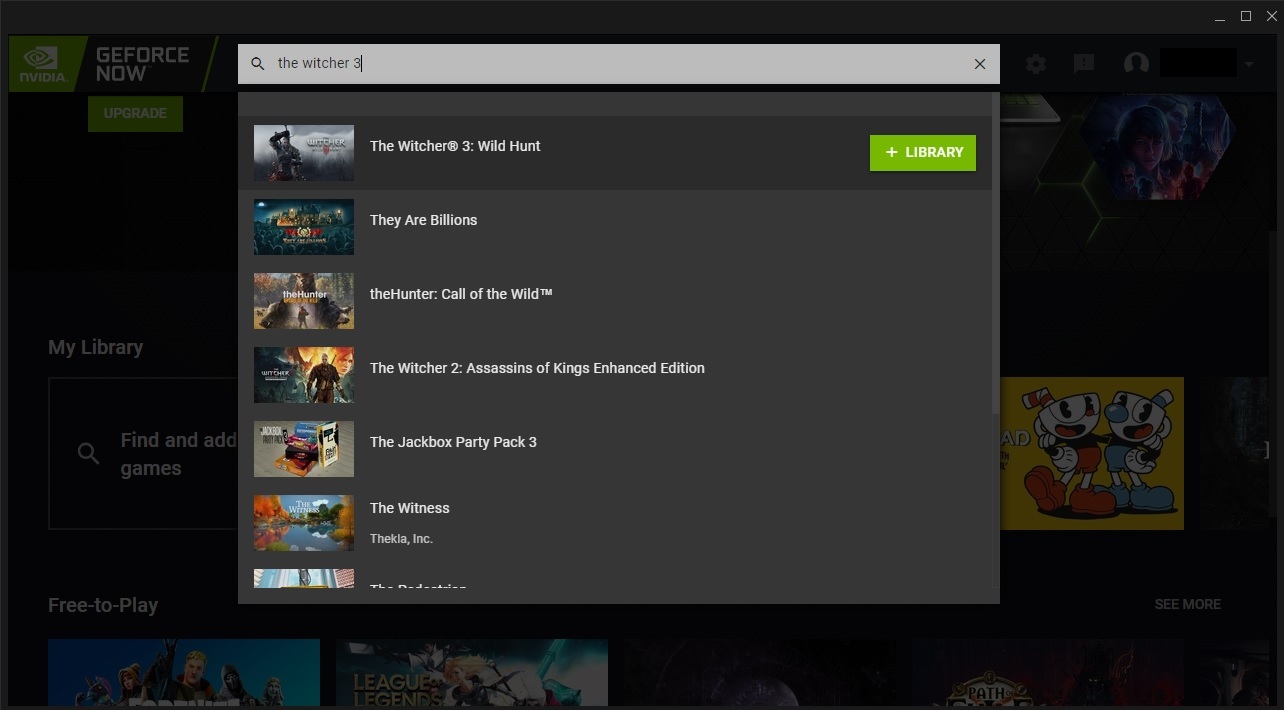The image showcases a user interface screen predominantly featuring a dark background filled with various content including images and text. A smaller, semi-transparent dark gray overlay box is present in the foreground, partially obscuring the main screen. At the top of this overlay box is a light gray search bar, where the user has entered the query "The Witcher 3." Below the search bar is a vertical list of game titles.

The first item in the list, "The Witcher 3: Wild Hunt," is highlighted in black. To its left, there is a thumbnail image of the game cover. To the right, there is a green button with the white text "Add to Library." The subsequent games listed below each have their respective thumbnails. These games are:
1. "They Are Billions"
2. "The Hunter: Call of the Wild"
3. "The Witcher 2: Assassins of Kings Enhanced Edition"
4. "The Jackbox Party Pack 3"
5. "The Witness"

The visible portion of the list ends here, with the image cut off, implying more entries might follow. In the background, the main screen shows additional game covers and related content.